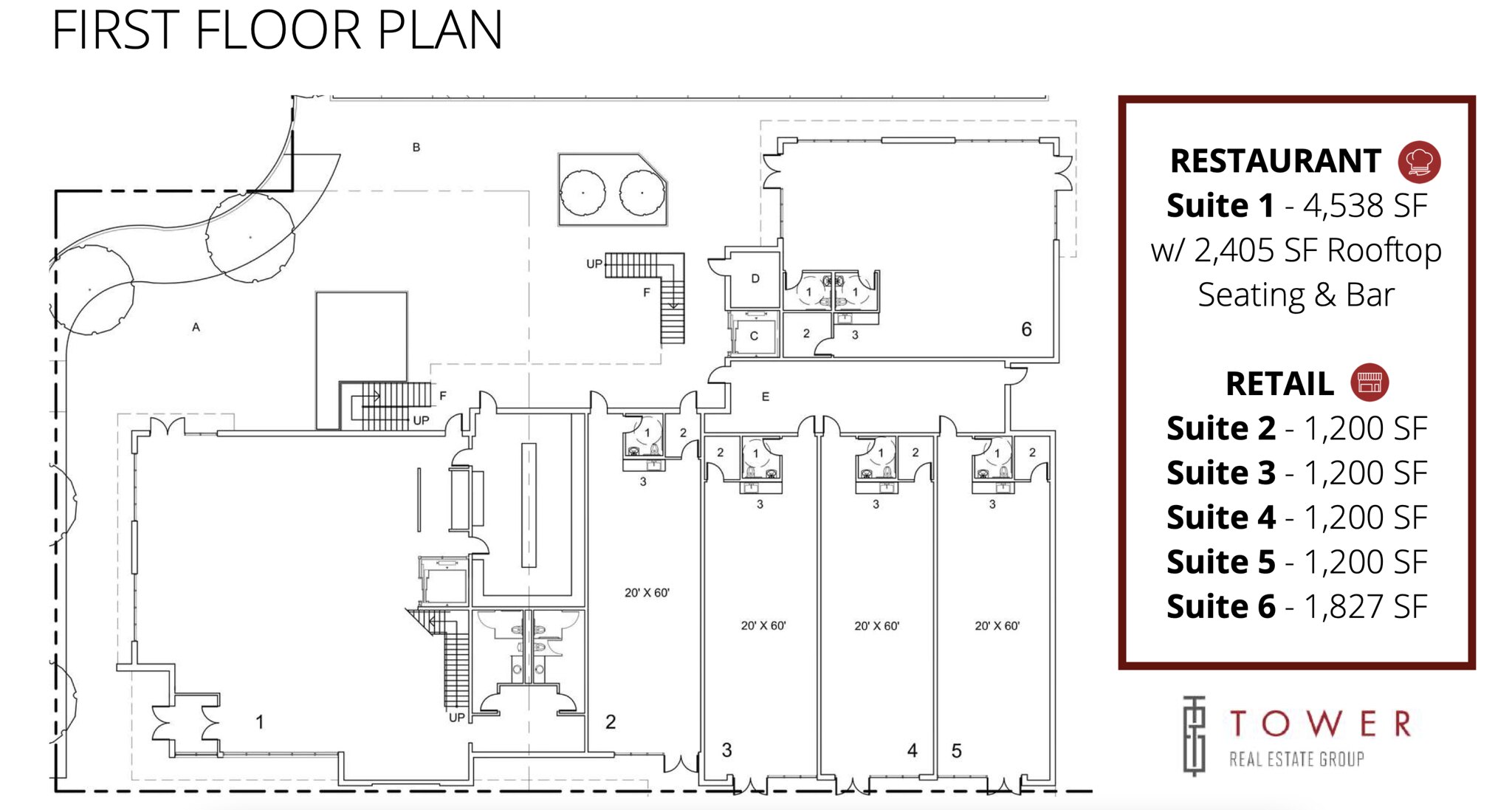The image is a detailed top-down view of a first-floor plan, illustrating both retail and restaurant spaces. To the right of the plan, there's a legend within a red-bordered square that categorizes and labels the various sections. Suite 1 is a restaurant encompassing 4,000 square feet, including an additional 2,000 square feet dedicated to rooftop seating and a bar, indicated by a small chef's hat icon. Adjacent to this are the retail spaces, labeled as Suites 2 through 6. Suites 2, 3, 4, and 5 each cover approximately 1,200 square feet, whereas Suite 6 is larger at 1,827 square feet. The floor plan visually segregates these suites: Suite 1 is positioned in the bottom left corner of the plan with a notable set of stairs, while Suites 2 to 5 line up beside it as elongated spaces. Suite 6 spans across a broader area, roughly equivalent to two and a half standard retail suites, and is situated opposite Suites 3 to 5. The bottom of the legend features the "Tower Real Estate Group," and the entire diagram resembles a map, offering a clear, organized depiction of the building's layout.